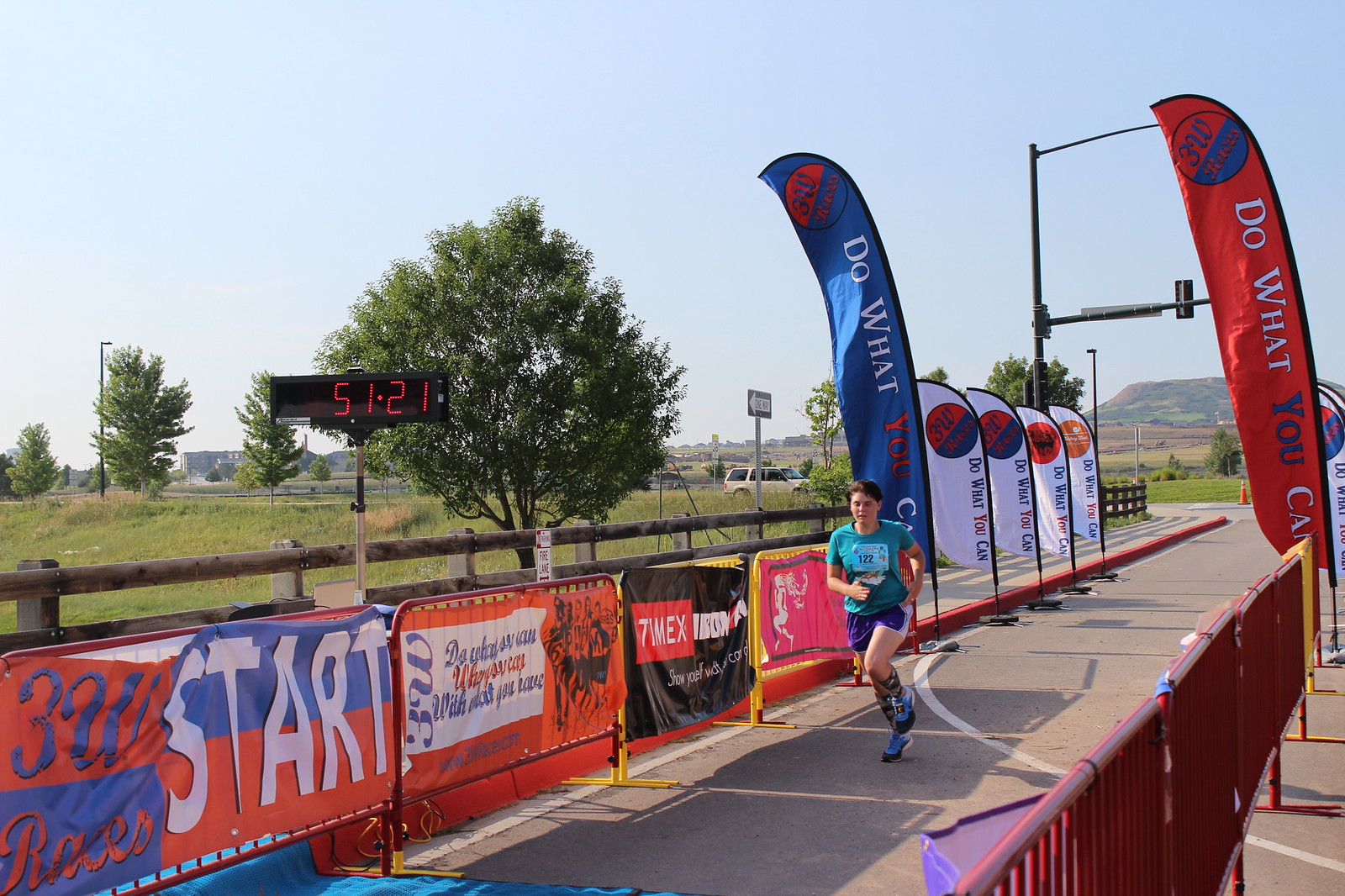The image captures a female runner nearing the finish line of a track and field race, set against a backdrop that suggests it might be in Southern California or Mexico due to the mountainous regions in the far distance. She is sporting a teal top and blue shorts with stripes, paired with blue running shoes. Her short hair flutters as she runs on a grayish-red track surface. To the left of the image, she is about to pass a digital clock on a pole displaying “51-21.” The track is lined with red barriers adorned with advertisements on both sides, marking the race path.

The left side of the image also features a wooden fence behind the barriers, with a grassy field and some trees visible. On the right side, behind the barriers, there are banners and street lights, along with cars parked near an intersection. In the distant background, beyond the guardrails, there are a few more trees, and the sky stretches out pale blue and cloudless. Tall blue and orange flags displaying the motivational phrase "Do what you can" line the path, contributing to the race's energetic ambiance.